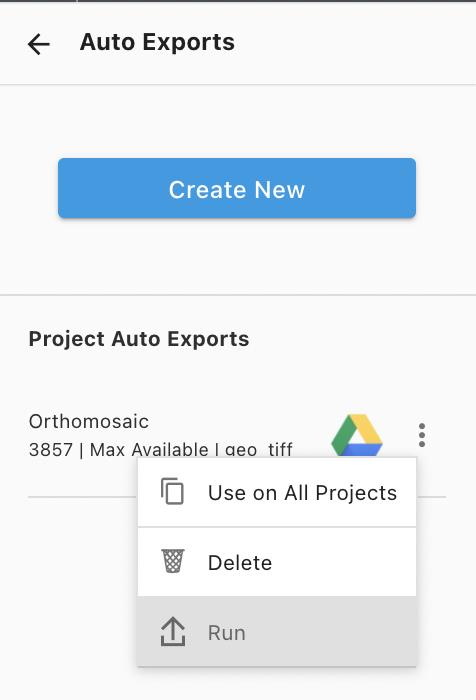In this screenshot with a light gray background, there is a thin black border at the top. Below the border, the bold black text reads "Auto Experts." An arrow points to the left, followed by a very light gray horizontal line. Beneath this line, a blue action button displays the text "Create New" in white. Further below, bold black text indicates "Project: Auto Exports," followed by smaller gray text listing details: "Ortho Mosaic 3857 Max Available GeoTIFF." To the right of this text, the Google icon is present. Below the Google icon, inside a white box, the text reads "Use on All Projects." Further down, the word "Delete" appears in dark gray text, accompanied by a trash can icon to the left.